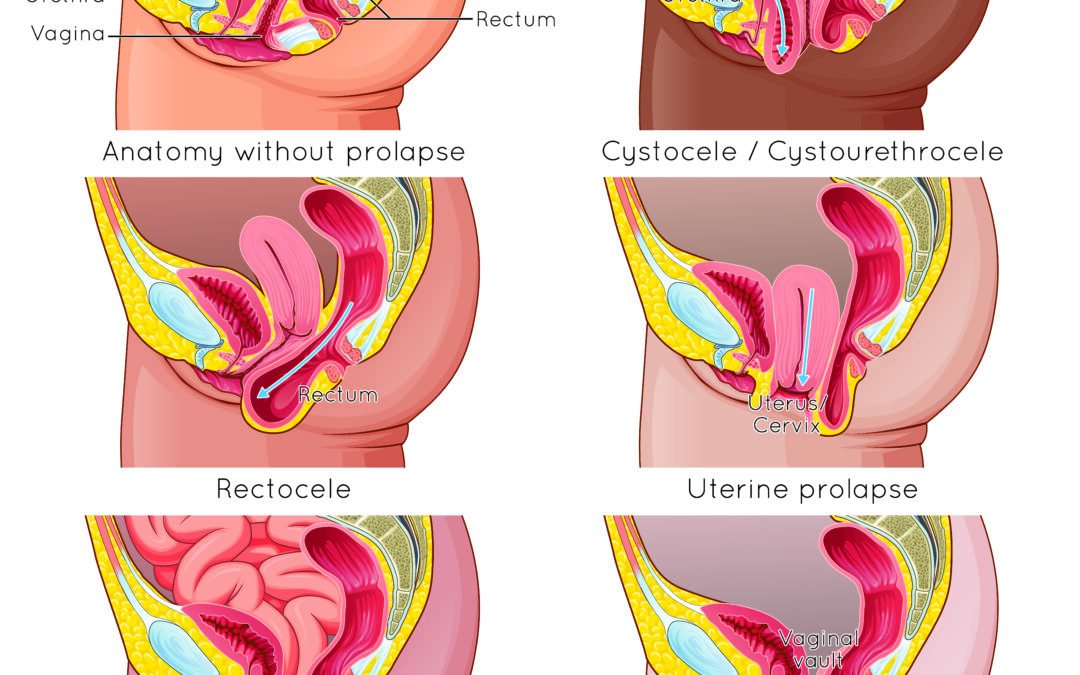This infographic from an anatomy and physiology book features colorful and detailed cross-sectional illustrations of a woman's pelvic region, highlighting conditions related to prolapse. At the top, black text labels identify various parts, including the vagina and rectum, which are depicted in dark pink tones. The rectum is shown along with yellow fat deposits, and a section with blue coloring, likely representing anatomical structures like the ovaries or other internal features.

The central images display comparative anatomy with and without prolapse. On the left, a diagram labeled "anatomy without prolapse" provides a clear view of the vagina, rectum, and adjacent organs. To the right, a similar illustration, accompanied by terms like "rectocele," "cystocele," and "cystourethrocele," shows how these structures appear when affected by prolapse conditions. Another image indicates "uterine prolapse," with a blue arrow pointing downwards at the prolapsed uterus and cervix. Pinkish depictions of the intestines are also visible in this comparative context.

The layout includes six total images, although four are partially cut off, limiting full visibility. Among these diagrams, one partially visible image is labeled "vaginal vault." Despite the truncation, the infographic effectively demonstrates the anatomy and medical conditions associated with pelvic organ prolapse, serving as a valuable visual aid in both medical training and understanding his condition's potential impacts.